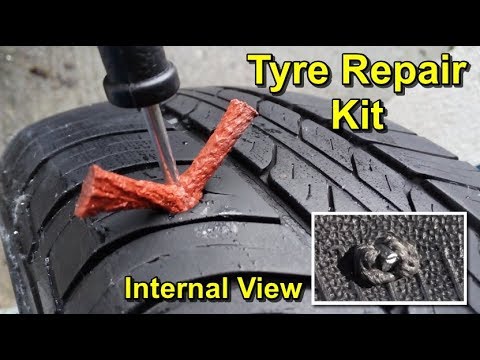This image resembles a still shot from a video, showcasing an advertisement or packaging for a tire repair kit. The screen is narrower due to black bars at the top and bottom. In the top right corner, there is yellow text with a black outline reading "Tire Repair Kit." At the bottom center, slightly smaller yellow text with a similar design states "Internal View." To the right of this text is a smaller, zoomed-in image with a white outline, which focuses on the damage to a tire.

The main image is a close-up of a black tire against a grey concrete background. Prominently featured is a tool with a black handle and a stainless steel silver shaft pressing an orange, polystyrene-like material into a V shape to seal a hole in the tire's center. The tire has a strong, well-defined tread and a thick central band. The tool appears to be inserting the material to stop a leak, indicating the function of the tire repair kit.